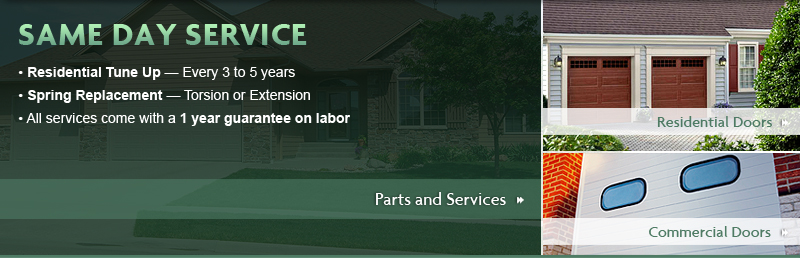This is a screenshot of a section of a website or banner. In the top left corner, "Same Day Service" is prominently displayed in green text. Below that, there is a bullet point list in white text. The list includes: 

- "Residential's Tune-Up," emphasized in bold, with a scheduling recommendation of every three to five years.
- "Spring Replacement," also in bold, followed by a note about torsion or extension.
- "All Services Come with a One-Year Guarantee on Labor."

Under the list, a green bar that states "Parts and Services" is visible.

The background image features a green-tinted photograph. On the left side of the image, there is a picture of the front of a brown house. On the right side, the image is divided into two sections. The top section, labeled "Residential Doors," displays two brown garage doors belonging to the house. The bottom section, labeled "Commercial Doors," showcases a white garage door with two blue windows.